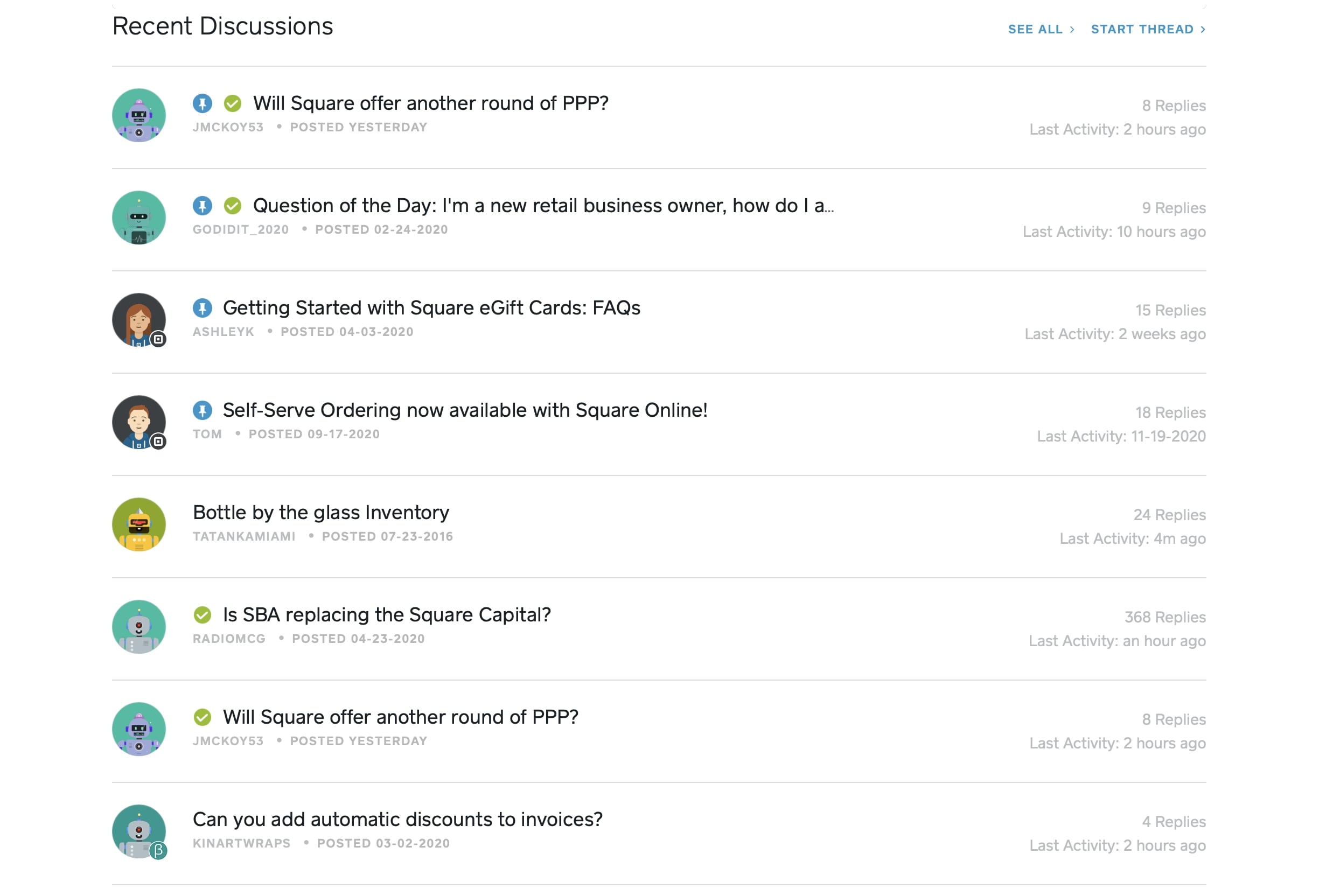This screenshot captures a webpage displaying a forum with various threads. The forum is titled "Recent Discussions," and it provides options to view all discussions or to start a new thread. There are eight discussion topics listed, each accompanied by a generic profile picture representing the post author, which include icons depicting a robot, a girl, and a boy rather than actual photos of individuals. The topics include:

1. "Will Square Offer Another Round of PPP?"
2. "Question of the Day: I'm a New Retail Business Owner, How Do I...?"
3. "Getting Started with Square E-Gift Cards: FAQs"
4. "Self-Serve Ordering Now Available on Square Line"
5. "Glass Inventory Management"
6. "Can You Add Automatic Discounts?"

The forum serves as a platform where users can post queries and participate in discussions related to Square's services and products.